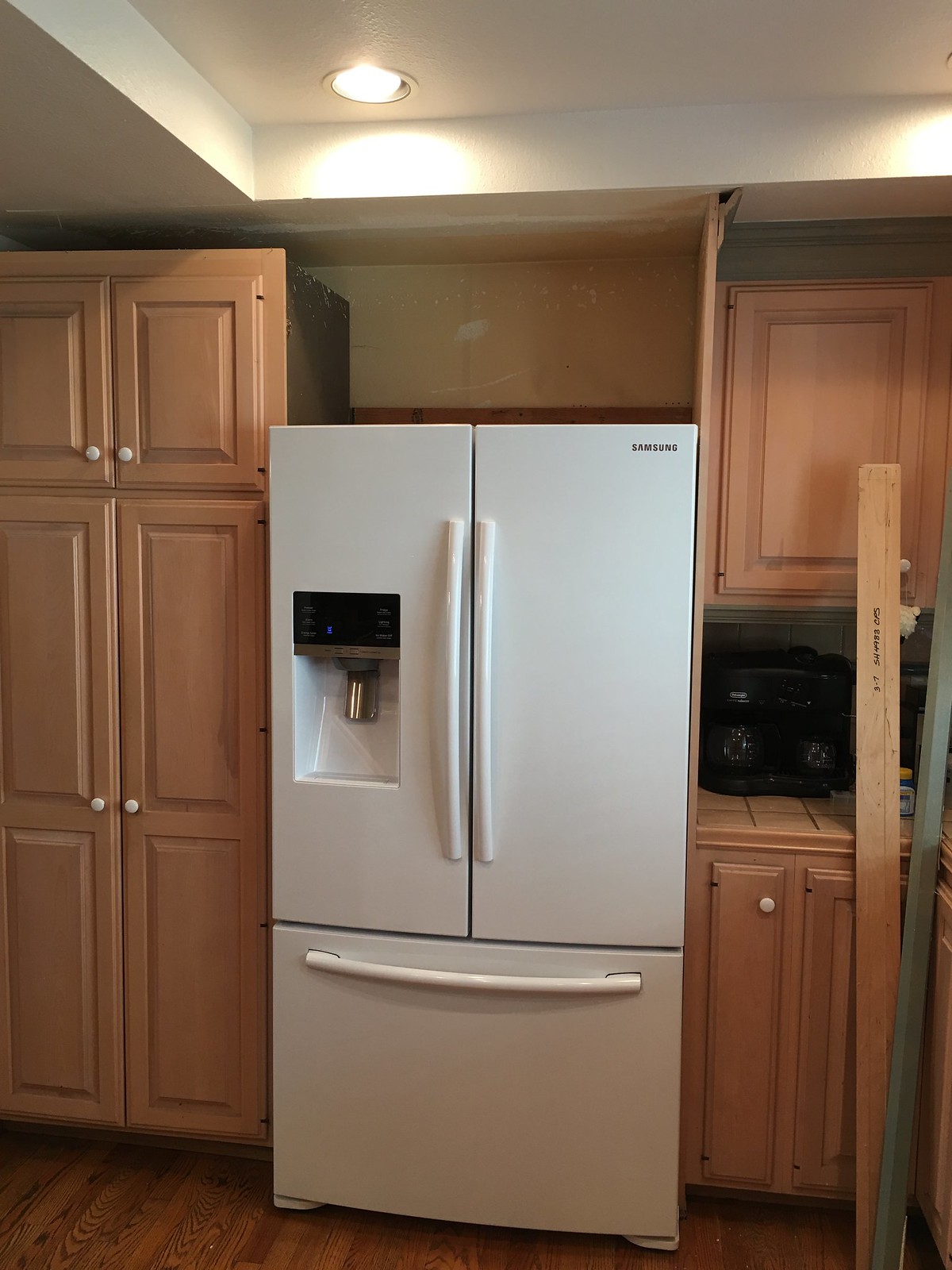The image is a color photograph taken inside a partially renovated kitchen, featuring a distinctive tray or coffered ceiling with recessed lights turned on. The kitchen cabinets are a pale pinkish hue, possibly unfinished or finished with a clear varnish, resembling light oak wood. Dominating the scene is a white Samsung refrigerator, set into an alcove between two stacks of cabinets—a floor-to-ceiling stack on the left and a countertop with both base and wall-mounted units to the right. The refrigerator has French doors at the top, a bottom pull-out freezer drawer, and an in-door ice and water dispenser with long white handles. Noteworthy is the blank space above the fridge, suggesting the kitchen is still undergoing construction, further evidenced by a piece of trim or floor molding standing in the corner. The floor is made of dark pine hardwood, and a black object, possibly a coffee maker or radio, is also visible.